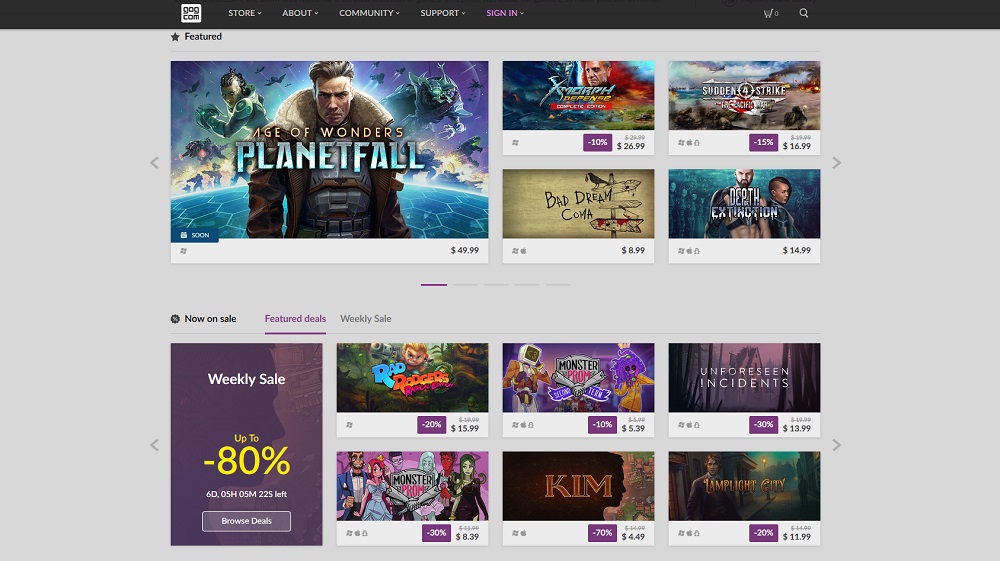The screenshot displays the main page of the website gag.com featuring a sleek black header with navigational options including "Store," "About," "Community," "Support," and "Sign In." Additionally, there are icons for the shopping cart and search functions.

Prominently displayed is a vivid promotional image for the game "Age of Wonders: Planetfall," showcasing a computer-generated character staring directly at the viewer. The character is donned in a dark brown leather jacket with underlying armor, alongside a price tag of $49.99.

To the right, an icon represents the game "Exmorph Defense Complete Edition," currently on a 10% discount, priced at $26.99. Below this, "Bad Dream: Coma" is notably illustrated with a sinister signpost, partially smeared with blood and topped by a crow, grasping a dangling object from its beak. This game is available for $8.99.

Following are discounts for other games: "Sudden 4 Strike" at 15% off, priced at $16.99, and "Depth of Extinction" priced at $14.99.

At the bottom of the page, the user has selected the "Featured Deals" section, displaying a countdown for the "Weekly Sale" which offers up to 80% off with six days, five hours, five minutes, and 22 seconds remaining. Notable discounted titles include "Rad Rogers" at 20% off ($15.99), "Munster Prom" at 30% off ($8.39), "Munster Prom Second Term" at 10% off ($5.39), "Kim" at 70% off ($4.49), "Unforeseen Incidents" at 30% off ($13.99), and "Lamplight City" at 20% off ($11.99). The section urges users to "Browse Deals."